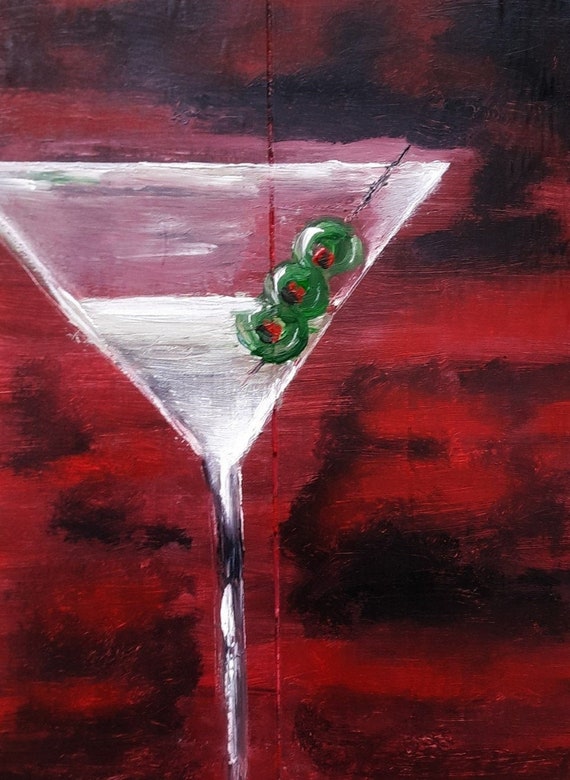The painting depicts a white martini glass, filled with a white-colored liquid, positioned against a striking background composed of alternating dark red and black strokes. The stem of the glass is prominently painted in white and black colors. Perched on the right side of the glass is a toothpick with three green olives, each featuring hints of white and red detailing. The olives rest diagonally and float on the liquid, secured by a black and white stick. At the top of the image, a pink streak of paint adds an additional layer of depth above the glass, while smudges of red and black paint around the edges contribute to the overall abstract and textured appearance. The base of the glass is not visible, as it extends beyond the canvas, adding a sense of intrigue to the composition.